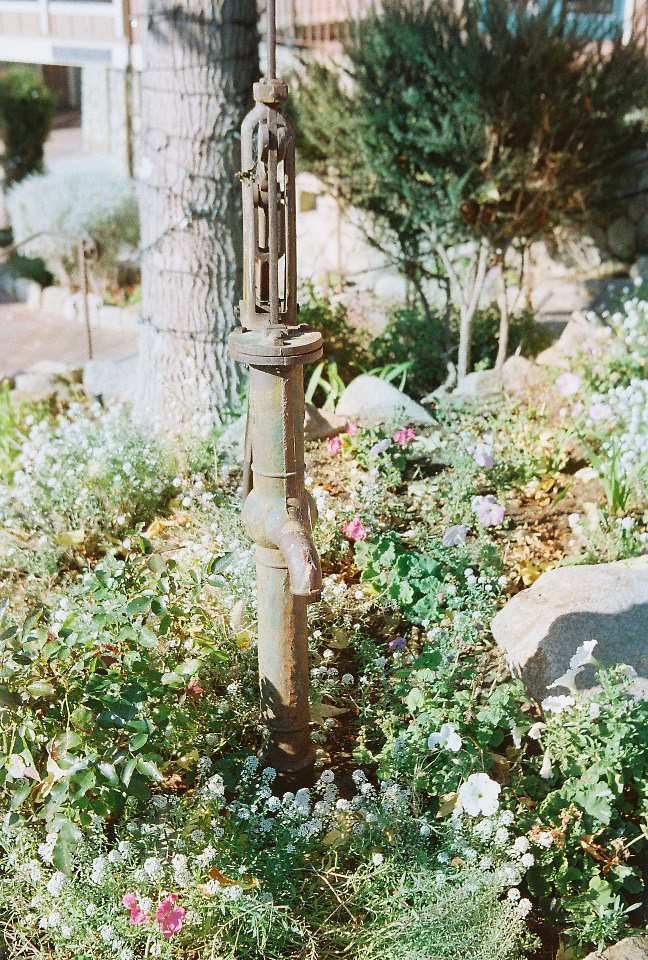The image captures a detailed view of an outdoor garden setting in the middle of the day, possibly near a small town. Dominating the lower portion of the image are various types of plants and vegetation, including grass, bushes, and flowers with occasional pink blooms among the predominantly green and brown foliage. Centrally placed is a slightly rusted, metallic water pump with a spout, surrounded by small bushes. The background features a blurred view of a plaza area with highly maintained small trees, some appearing pale and others with green and brown leaves. To the top left, a partial view of a brick walkway is visible along with additional trees and buildings, and there appears to be an archway that leads to more vegetation and trees. The overall palette includes tan, white, black, green, pink, dark green, and brown shades, enhancing the natural, rustic charm of the garden scene.